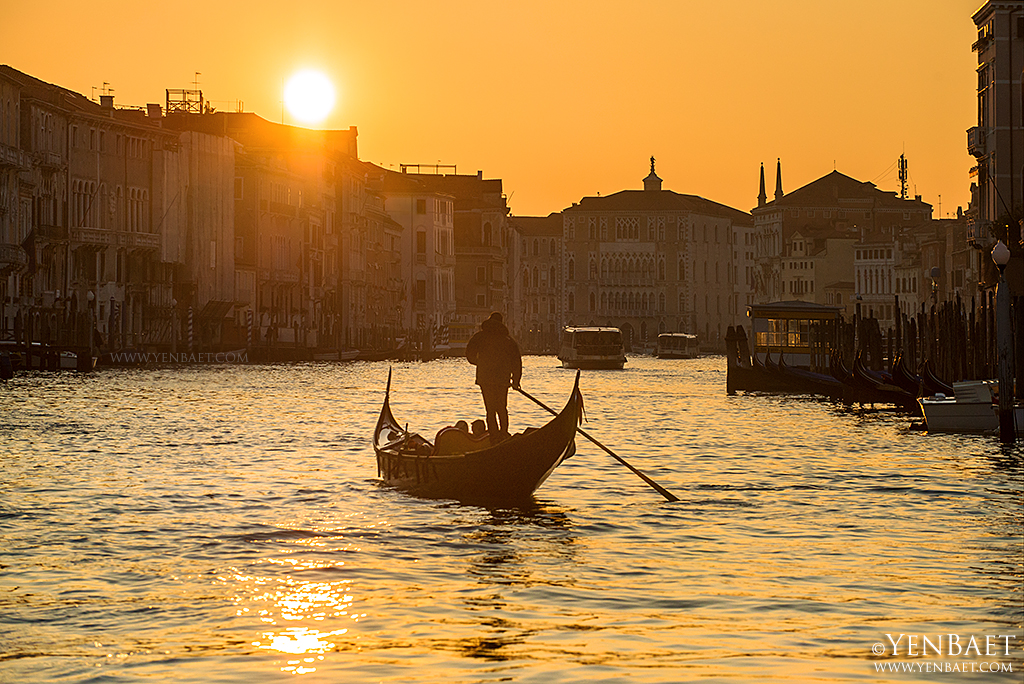This photograph, shot outdoors likely around sunset, captures a picturesque canal scene with a warm, yellow sky and a brilliant orange hue. The sun, either rising or falling, is a bright white circle positioned over a building on the left side. The bottom half of the image features a canal stretching from left to right, with a combination of blue and yellow reflections in the water. At the center of the canal, a gondola is steered by a man standing and rowing, with people seated in front of him. The gondola, tilted slightly to the left, leads away from the viewer.

Flanking the canal on both sides are multi-story stone buildings with tan facades and white accents around the windows and doors. Their roofs are predominantly brown, some adorned with pointed structures and chimney-like features. The backdrop is decorated with white light posts and a series of red and white striped poles along the docks. In the distance, several pontoon boats and unoccupied blue boats are visible near the shore, alongside white boats, some with yellow markings.

At the bottom right corner of the photograph, there is a copyright symbol (©), followed by the text "YENBAET" in large, all-capital letters, and underneath in smaller letters, "www.yenbaet.com," all in white print.